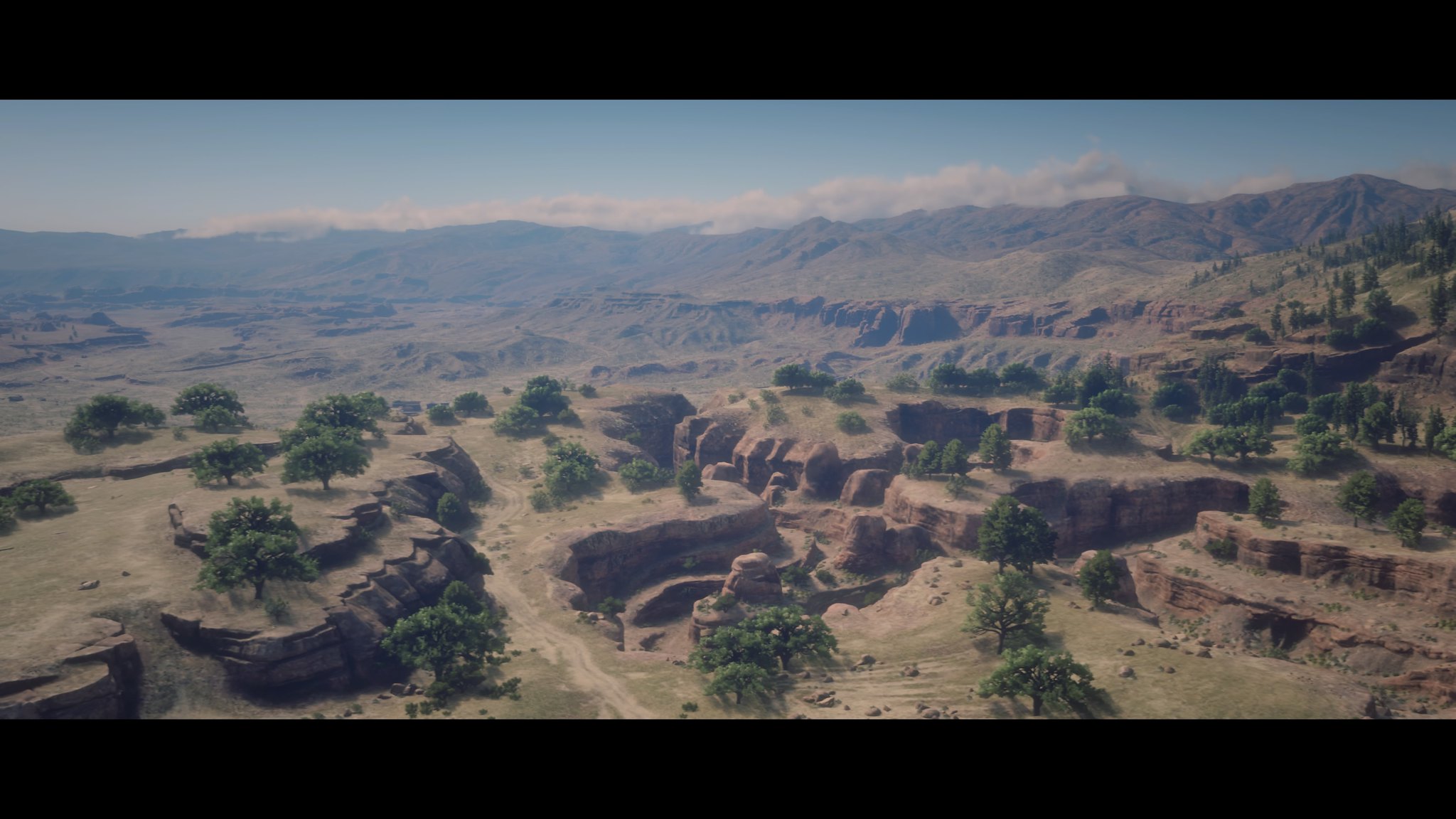This panoramic image captures a breathtaking, wide-angle view of a mountainous landscape. In the distance, a rugged mountain range stretches across the horizon, with wisps of clouds clinging to its peaks and a clear, azure sky above. The foreground reveals a network of dirt roads and trails meandering through a highly eroded, brown terrain marked by various shades of tan and darker earthy tones. Trees sporadically dot the tops of buttes and small canyons, adding contrast to the otherwise arid scenery. The eroded formations display smoothly rounded contours from their summits to their bases, illustrating the forces of nature that have shaped this land over time. The image likely captures a scene from the western United States, characterized by its distinctive erosion patterns and sparse vegetation amidst an expansive, dramatic setting.